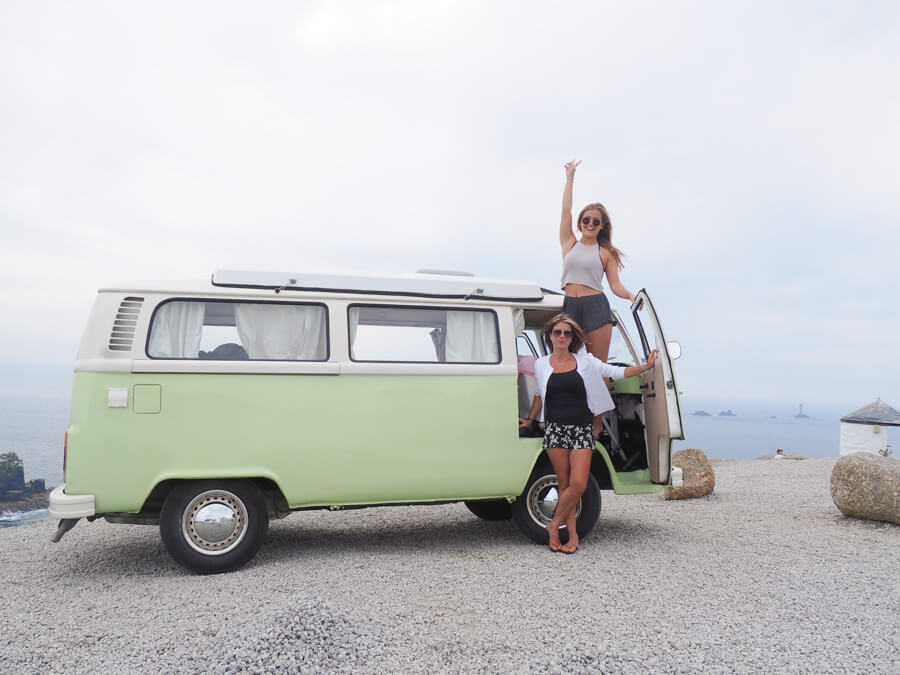In this vibrant vacation photo, two young women, likely in their late teens or early 20s, are posing in front of a vintage 1960s-style Volkswagen bus. The bus, painted a light, creamy green with a white roof and window trim, is parked on a gravel area overlooking the ocean, with large rocks preventing access to the beach. The backdrop includes a cliff face and distant ships on an overcast day.

The woman standing in front of the bus on the ground wears black and white shorts, a black top, and a stylish white long-sleeved jacket. She has sunglasses on and her blonde hair cascades just below her shoulders. Beside her, another woman stands elevated on the bus ledge, barefoot and dressed in gray shorts and a white tank top, exposing her midriff. With her long hair flowing, she too wears sunglasses, capturing the carefree spirit of the moment by flashing a peace sign. This picturesque scene captures the essence of coastal adventure and youthful exuberance.